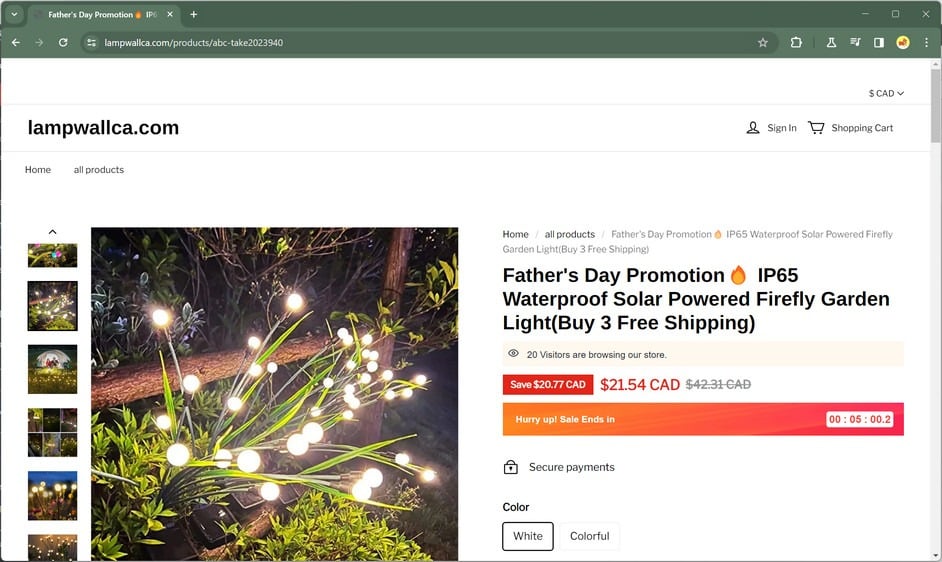This is a detailed screenshot of a promotional web page from the Canadian online store lampwallca.com, featuring a Father's Day offer. The page prominently advertises an IP65 waterproof, solar-powered firefly garden light with a little fire emoji emphasizing the hot deal. Customers can take advantage of an offer where purchasing three lights results in free shipping. Below the product description, a live indicator shows that 20 visitors are currently browsing the store.

A call-to-action button in red attracts attention with the text "Save $20.77 CAD." The original price of $42.31 CAD, now crossed out, highlights the discounted price of $21.54 CAD. Urgency is added with a banner stating "Hurry up, sales end in five minutes." To assure customers, the message "Secure payments" is displayed.

The web page also provides choices for the light's color options—white or colorful. At the top navigation bar, users have options to go back to the homepage, view all products, sign in, and access their shopping cart. Additionally, the top right-hand corner of the page allows users to select the currency type, which is currently set to CAD.